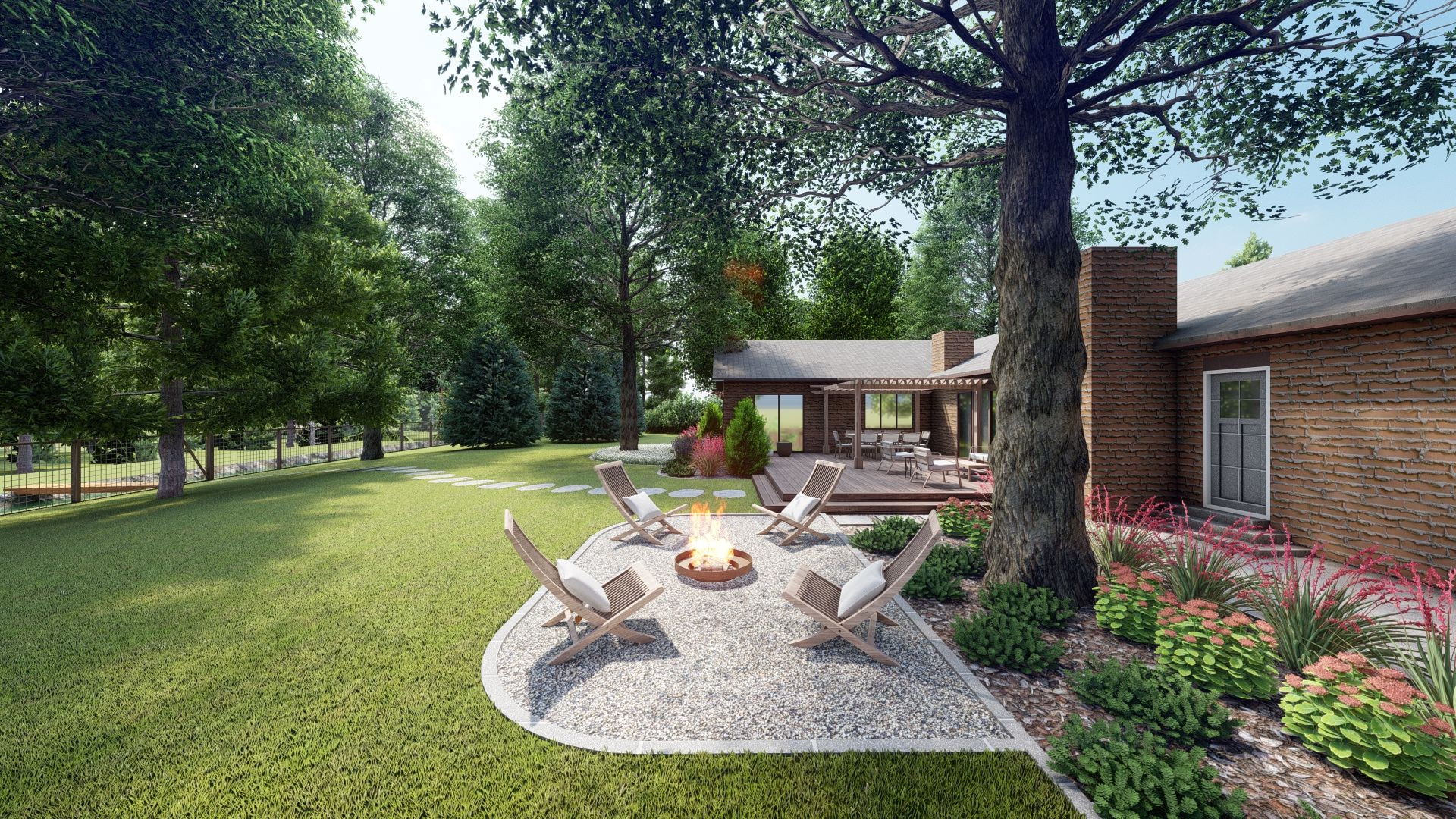This horizontal-rectangular image showcases the meticulously maintained backyard of an upper middle-class, 1950s-style, one-story brick home with a gray roof. The focal point is an expansive, lush green lawn, bordered by an impressive row of mature trees along a sidewalk at the back. Central to the yard is a wooden deck adorned with various white patio furniture, including chairs and tables, all sheltered by a tall wooden awning. Adjacent to the deck, a stone pathway leads to an oval-shaped gravel area with a bordering gray brick, featuring a fire pit with an active fire and four lawn chairs facing each other. The garden area, abutting the house, displays an assortment of plants complemented by a distinct white stone section, adding to the backyard's charm. This serene and aesthetically pleasing setting might be mistaken for a 3D rendering due to its near-perfect staging, potentially arranged for a real estate presentation.